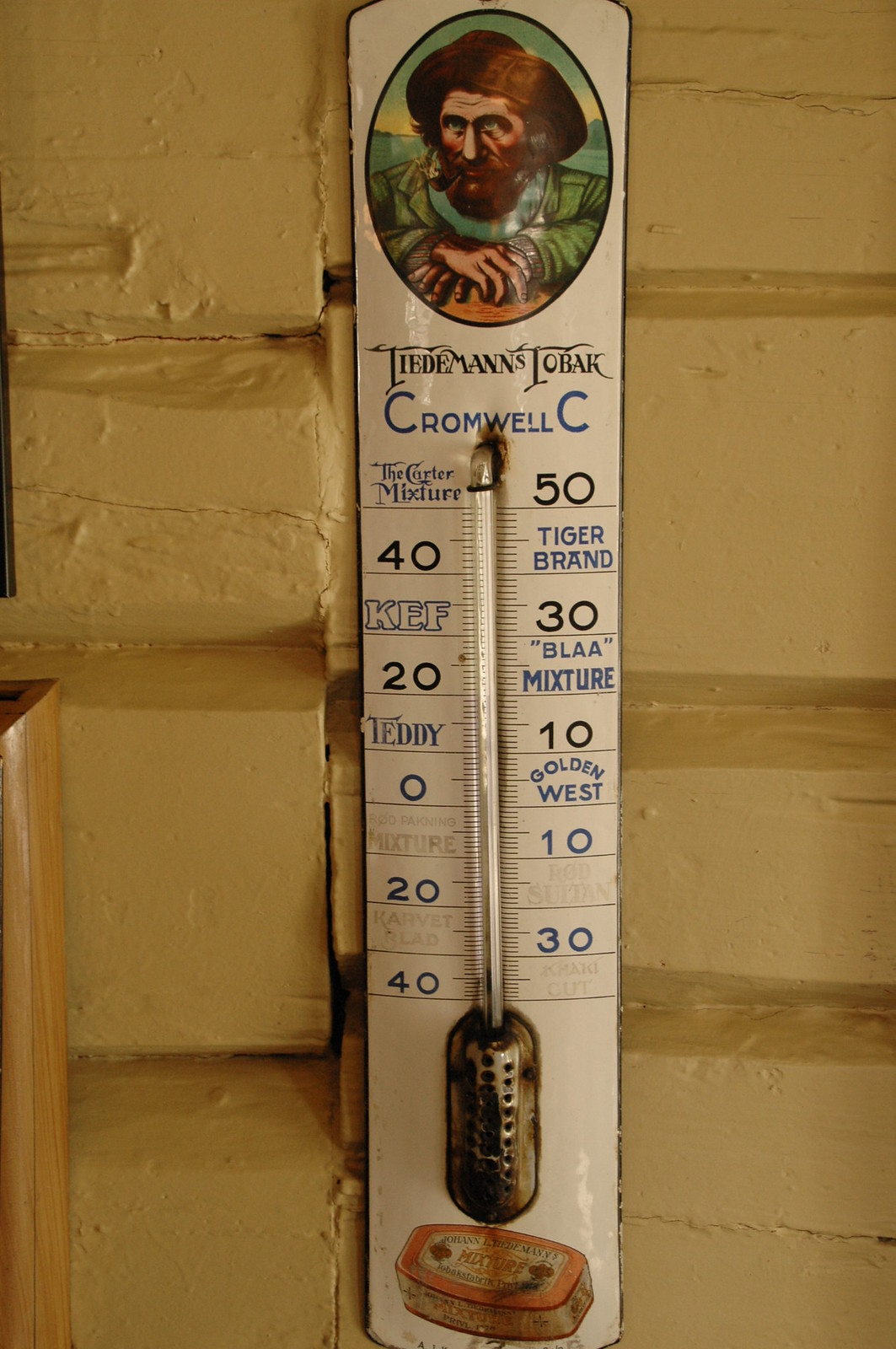A vintage-style metal thermometer hangs on a beige-painted wooden wall. The thermometer itself is white with distinct features. At its top, there is an oval portrait of a man with brown hair and a beard, wearing a green shirt. Below the portrait, the inscription reads "Tideman's Toeback, Cromwell C." The central portion of the thermometer contains a clear tube with metallic components—a small metal section at the top and a pill-shaped metal element at the bottom, indicating temperature. Alongside the thermometer, numerical values in blue text range from 40, 20, 0, -20, to -40, and back up to 50, 30, 10, -10, and -30. Each number is paired with text, including brand names and mixtures such as "Tiger Brand," "Teddy," "Golden West," "Kef," "The Carter Mixture," and "Blah Mixture."